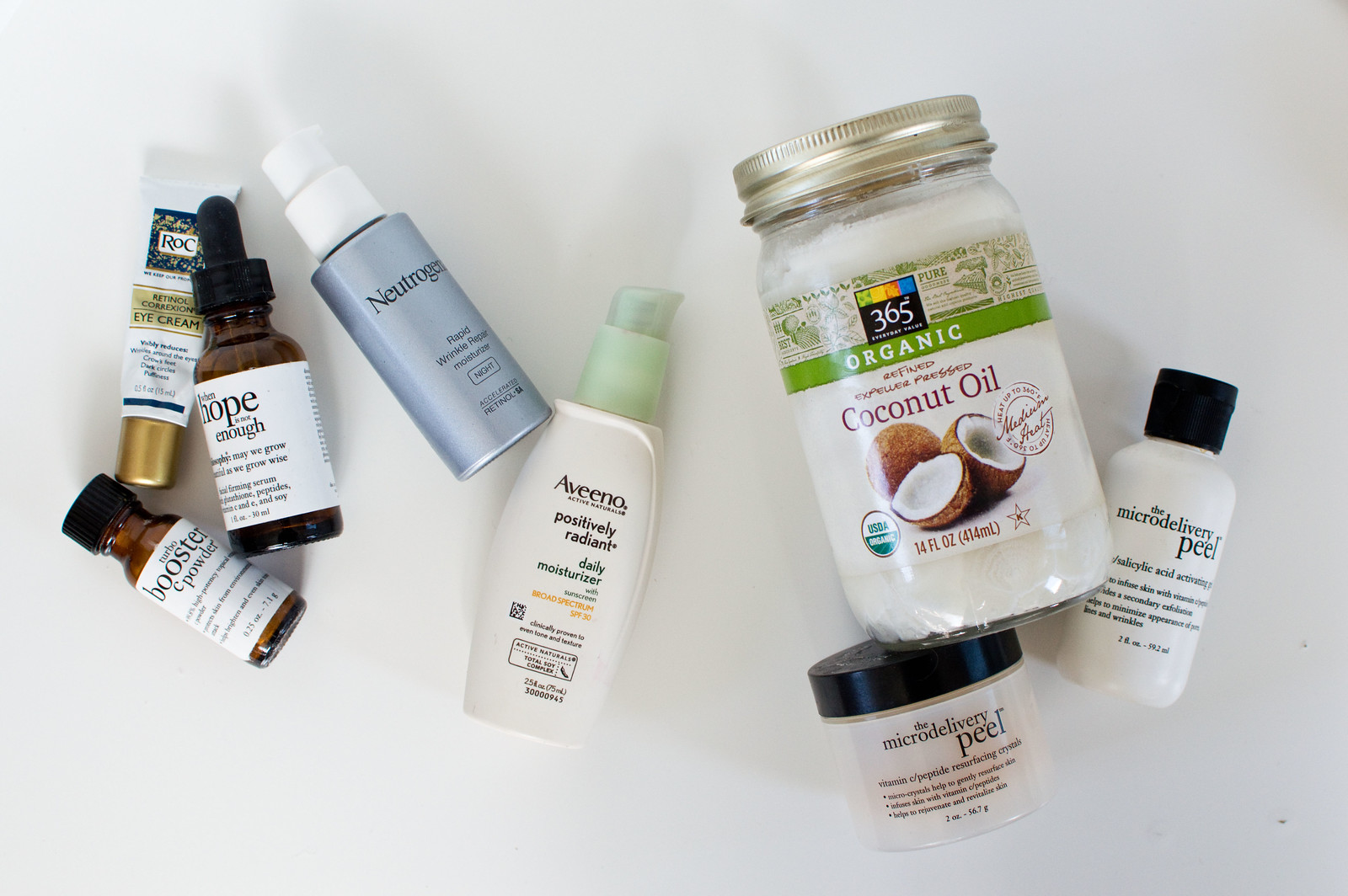In the image, a collection of various skincare and face products is meticulously arranged on a pristine white countertop. The assortment includes an eclectic mix of bottles, jars, and containers, each serving a unique purpose in a skincare regimen. 

On the far right, a prominent jar labeled "Organic Coconut Oil" stands out with its vividly illustrated label featuring two coconuts, one of which is split open to reveal its interior. This product is likely heralded for its natural moisturizing properties.

Towards the bottom of the display are two items from the same product line, "Micro Delivery Peel." One is housed in a tall bottle while the other resides in a shorter container, both essential components of a comprehensive exfoliating routine.

On the left side of the image, two sleek, dark glass bottles capture attention. One is identified as "Booster Powder," a likely candidate for boosting the efficacy of other skincare products, while the other is labeled "Hope Enough," which might be a nourishing serum or elixir. Nestled beside these is a modest-sized eye cream with "Roc" prominently displayed at the top of its label, suggesting targeted treatment for the delicate skin around the eyes.

Centrally positioned are two familiar brand-name products, indicating their widespread use and accessibility. One bottle showcases the "Aveeno" brand, known for its gentle, soothing formulations, while the adjacent "Neutrogena" product is likely celebrated for its dermatologist-recommended solutions.

Overall, the image presents a varied selection of skincare essentials, each carefully placed to highlight its unique contribution to a well-rounded beauty routine.